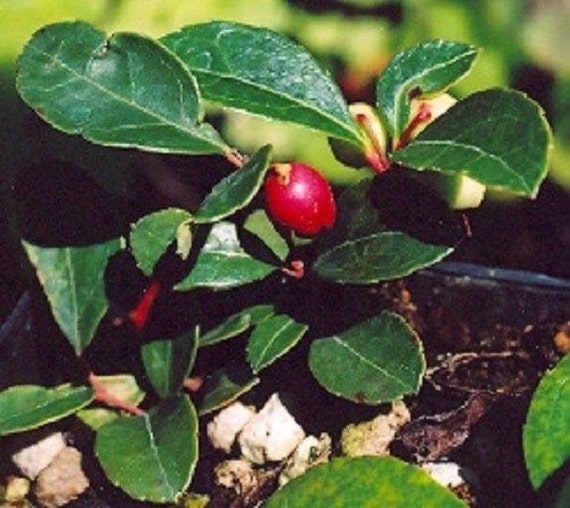In this image, a green plant takes center stage, dominating the frame with its vibrant foliage. The leaves are narrow and oblong, resembling teardrops, with notable veins and a faint reddish tint along the stems, especially visible in the upper right. Nestled among these leaves is a striking red berry, oval-shaped and deep in color, suggesting ripeness. Another berry, however, appears light yellow to green, hinting it might not be fully matured yet. The foreground reveals white rocks scattered on the soil, which transitions into darker brown dirt at the plant’s base. The background, blurred and out of focus, suggests the setting is an outdoor garden or a natural environment, devoid of any text or human presence. The grainy quality of the image implies it is an older photograph.